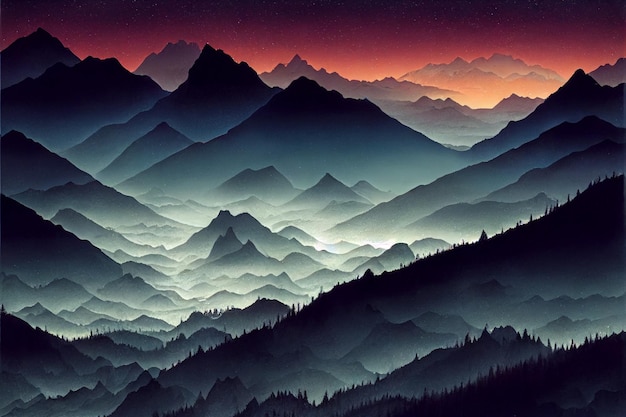The image is a captivating digital artwork depicting a vast, hilly, and mountainous landscape. The scene is painted with a dramatic and contrasting color scheme, blending warm and cool tones. At the upper part of the image, the sky transitions from almost black to deep reddish-orange hues, indicative of a recent sunset. Dark, triangular mountains dominate the horizon, casting a stark contrast to the vibrant sky. 

In the foreground, rolling hills stretch extensively into the distance, skewed slightly to the left. These hills start black at their peaks, adorned with the silhouettes of sharp, pointy pine trees, and gradually transition through dark grey to light white in the middle portion of the image. 

The middle ground features particularly hilly areas illuminated by an enigmatic white light emanating from the ground, without any visible light source. The smaller hills and mountains here appear to be enveloped in swirling clouds, adding to the surreal atmosphere of the scene.

The overall landscape, draped in this interplay of light and shadow, showcases a spectrum of colors—warm reds, oranges, and purples in the upper sections blending into cooler blues and whites below—creating a striking and beautiful portrayal of nature.